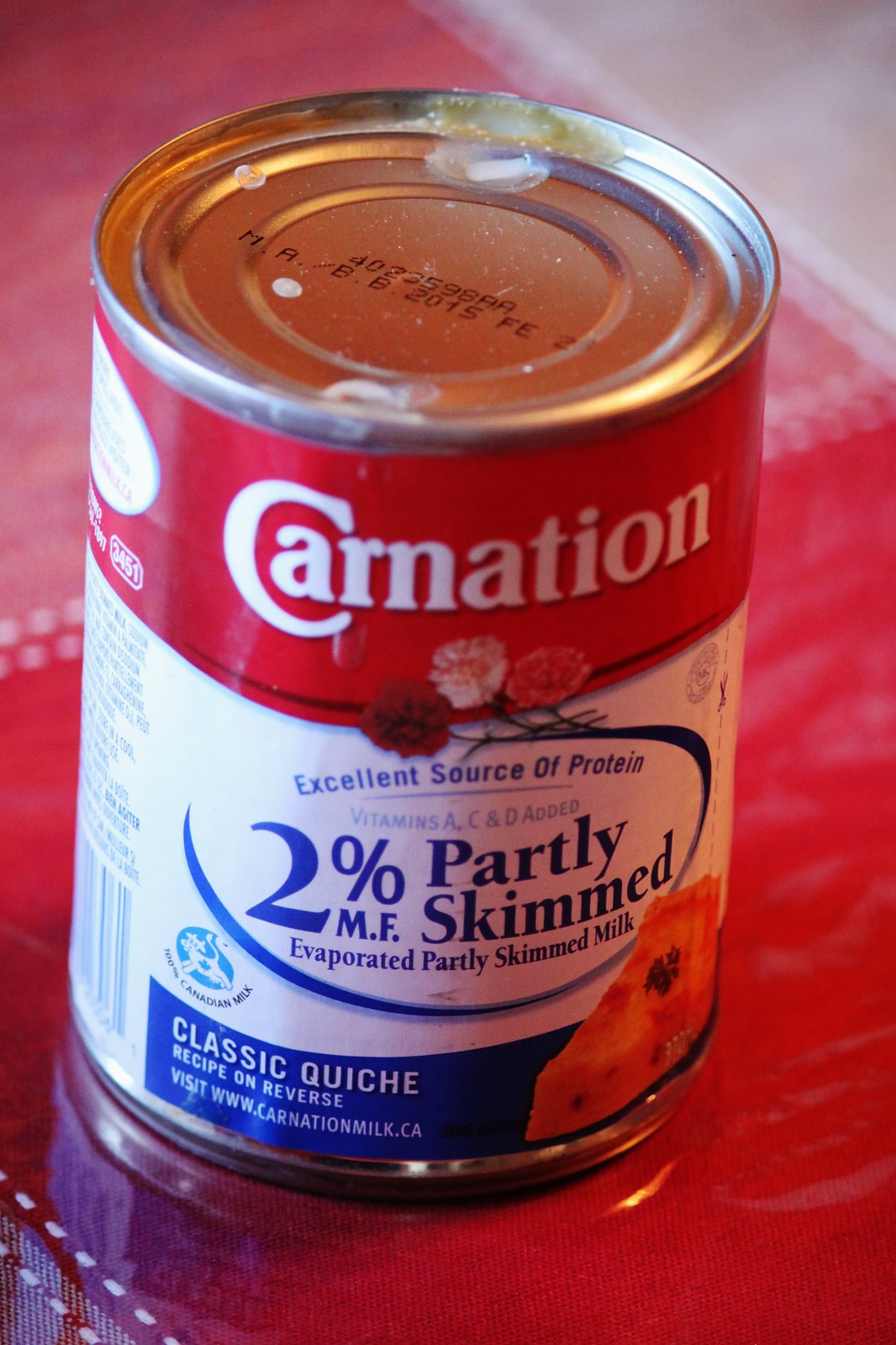A close-up photograph captures a well-used can of Carnation partly skimmed evaporated milk, prominently featuring its distinct red, white, and a touch of blue color scheme. The can's lid has been opened on both ends, revealing remnants of solidified or crusted milk at the top. The Carnation logo is clearly visible, along with an image of three blooming carnation flowers. The label details that this product is an excellent source of protein and is fortified with vitamins A, C, and D. It specifies that the milk contains 2% milk fat. Towards the bottom of the label, there is an advertisement for a classic quiche recipe available on the reverse side, as well as a website URL, www.carnationmilk.ca, indicating its Canadian origin.